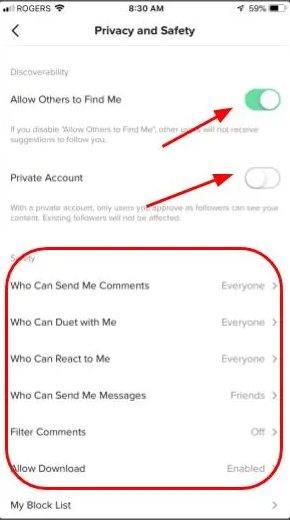This image, captured at 8:30 a.m. with a 59% battery and two bars of Rogers network signal, displays the "Privacy and Safety" settings screen. At the top left, there’s a back arrow, indicating navigation. Below, the "Discoverability" section is featured prominently with a green toggle switch for "Allow others to find me," emphasized by a red arrow. The "Private account" option is turned off, highlighted by another red arrow. Subsequent sections detail various settings: 
- "Who can see my comments" set to "Everyone"
- "Who can duet with me" set to "Everyone"
- "Who can react to me" set to "Everyone"
- "Who can send me messages" set to "Friends"
- "Filter comments" set to "Off"
- "Allow downloads" enabled
- "My block list"

The important sections are circled in red for emphasis.